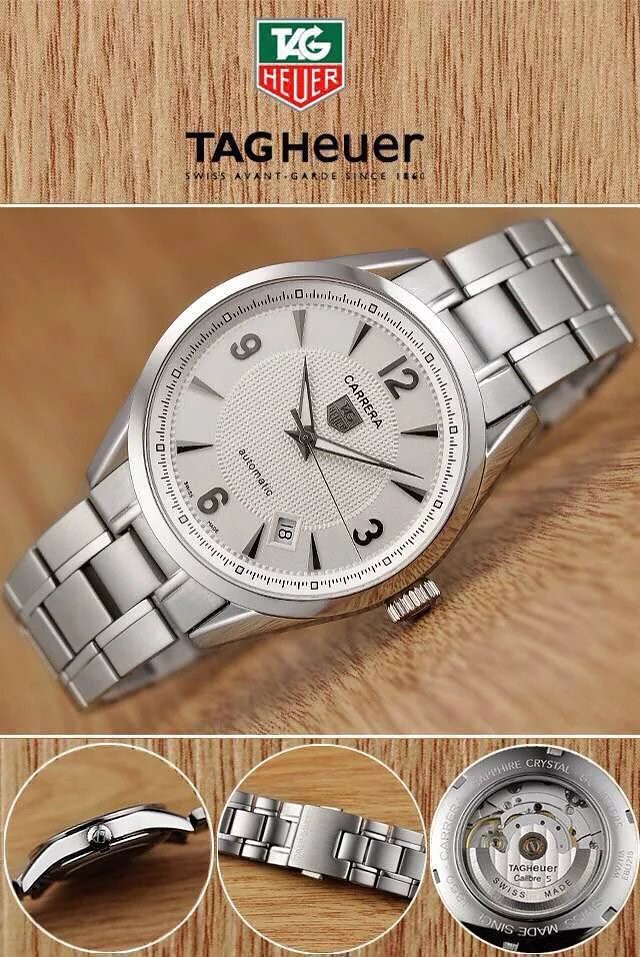Advertisement for TAG Heuer Carrera Wristwatch:
 
This detailed advertisement features a sophisticated TAG Heuer Carrera wristwatch set against a vertical wood grain background, accentuating the classic elegance of the design. Dominating the foreground, the bright silver watch has a round face with prominent markers at the 12, 3, 6, and 9 positions, interspersed with sleek slashes for hour markers. The watch face itself is a blend of metal and a pale center, complemented by a metal band. The TAG Heuer logo, characterized by a green upper half and a red lower half, appears at the top of the image, with the words "TAG Heuer" in bold black letters beneath it. An additional inscription on the watch reads "Carrera," further emphasizing its high-end brand.

Beneath the main image, three circular close-up shots provide an in-depth view of the watch's craftsmanship. From left to right, these zoomed-in images showcase the side of the watch with its intricate knob, the precise clasp mechanism of the band, and the intricate inner workings of the timepiece.

The seconds on the watch face are subtly visible in the central angle, adding to the precise detailing. The overall composition, from the rich wood grain background to the polished silver watch, highlights the luxurious and avant-garde sense that TAG Heuer is renowned for.